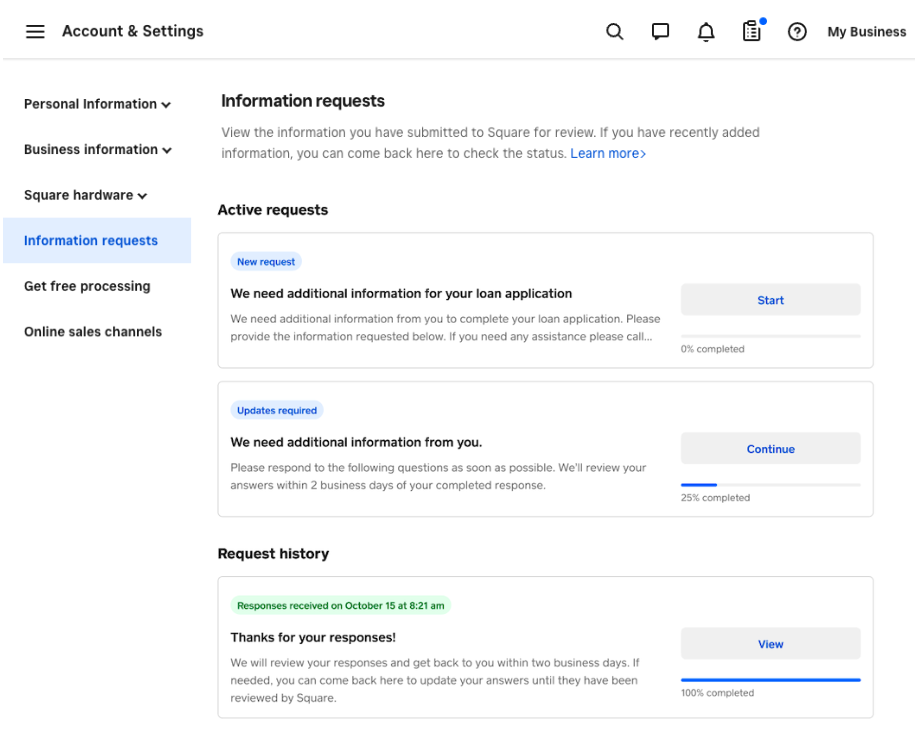The image showcases a comprehensive account management webpage. At the upper left-hand corner, the section labeled "Account and Settings" is prominently displayed. Above this, a hamburger icon consisting of three lines is positioned for easy navigation. On the right-hand side of the header, the navigation elements begin with "My Business." Moving leftwards from here, there is a circle containing a question mark, followed by an icon resembling a clipboard with a blue dot on top. This sequence continues with a bell icon, a comment icon, and a search icon.

Directly below the "Account and Settings" section, a horizontal line separates the header from the main content area. The sidebar features options such as "Personal Information," "Business Information," and "Square Hardware," each equipped with drop-down arrows for expanding further details. "Information Requests" is highlighted in gray with blue font, indicating its active status. Beneath this, a promotional message reads, "Get Free Processing Online Sales Channels."

In the central part of the page, the words "Information Requests" are prominently displayed again, followed by a detailed body of information. This section also features a subheading labeled "Active Requests," under which three rows of requests are listed:

1. "We need additional information for your loan application," accompanied by a "Start" button.
2. "We need additional information from you," accompanied by a "Continue" button, and below this, "25% complete" is indicated.
3. "Request History" is the heading for the next section, which contains an entry stating, "Thanks for your response," alongside a "View" button. This entry is marked as "100% complete."